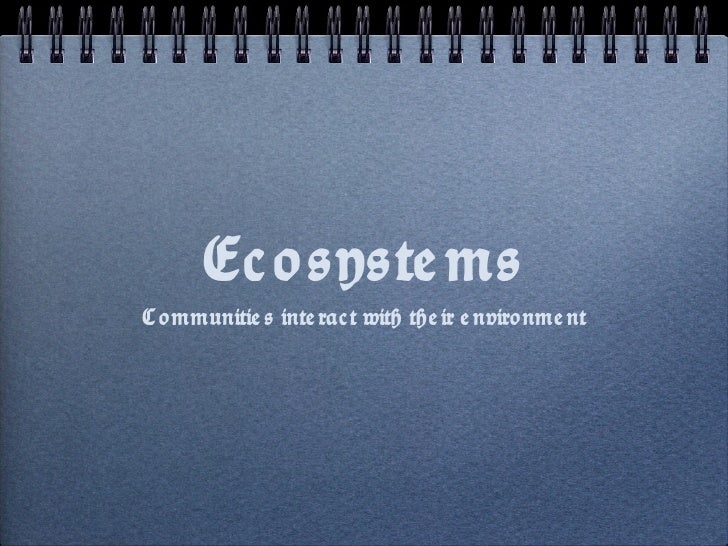The photograph captures a spiral-bound notebook placed on a black surface. The notebook, which occupies nearly the entire frame, features a textured blue cover that appears to be made of a sturdy paper-like or cardboard material. At the top of the cover, a metal spiral binding is visible, threading through square holes to hold the pages together. The focus of the image is the cover's white text, with the large title reading "Ecosystems" at the center, followed by a smaller subtitle, "Communities interact with their environment." The text is neatly centered, contributing to a well-balanced and aesthetically pleasing composition. Despite the classic printing style, there are noticeable gaps between some of the words, giving it a distinctive yet slightly unconventional appearance. The overall style of the notebook is elegant, suggesting it could be used in both educational and professional settings. The colors in the image include shades of blue and white on the notebook, contrasted by the dark background.